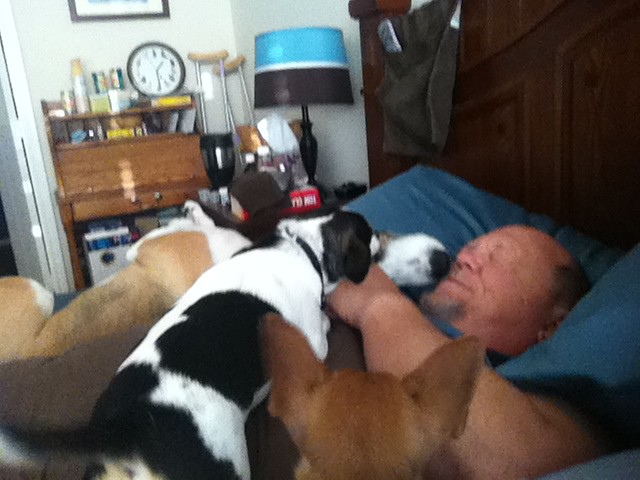This photograph captures a detailed bedroom scene where a man, who is balding with some gray hair and a gray goatee, is lying in bed. The bed features a dark wooden headboard, blue sheets, and a blue pillow under his head. His eyes are squinted shut, possibly in pain or discomfort, and several dogs surround and console him. At least three dogs are clearly visible: a black and white dog is lying on top of him, licking his face; the back of a brown dog’s head is seen near the lower center of the image, and a tan and white dog is sprawled out sleeping near the bed's edge.

The room itself is neat but filled with various items. A turquoise and brown lamp with a dark brown base stands out against the tan-colored walls. A writing desk, cluttered with a clock, some spray, and a couple of boxes, is visible alongside a small dresser and crutches leaning against the wall. A red object rests on the nightstand beside him. Hanging over the bed is a remote control holder. There's also an open door on the right edge of the picture and an unidentifiable image hanging on the wall. The scene paints a picture of a cozy, lived-in space with the man receiving affection and care from his dogs amidst his apparent injury.